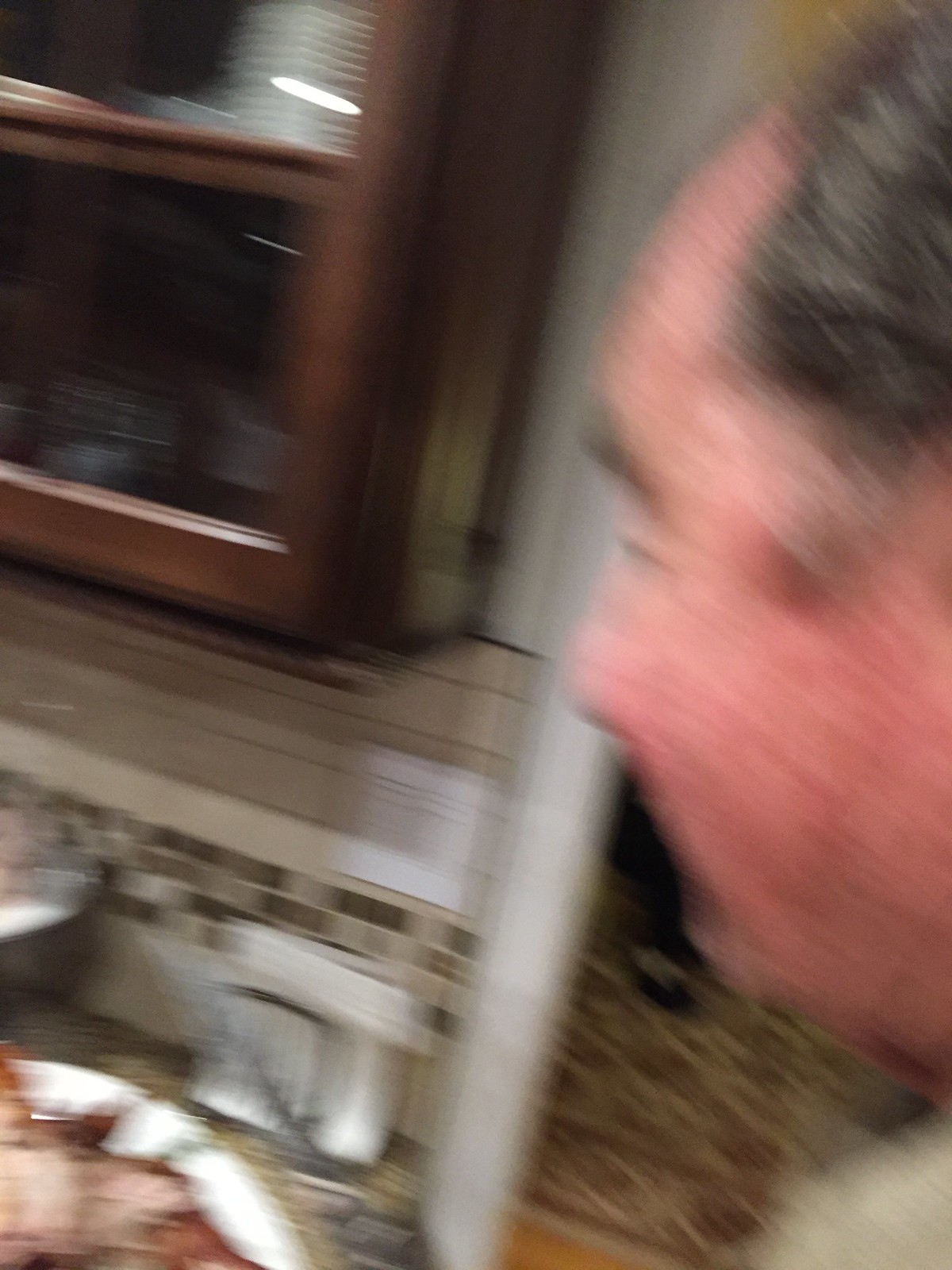A blurry close-up image captures a gray-haired man walking into the frame from the right, facing left, within a kitchen setting. The left side of his face and a small portion of his shoulder are visible in the shot. The background reveals kitchen cabinets, a countertop, and a backsplash wall. In the lower left corner of the image, a plate with what appears to be pizza is partially visible on the countertop.